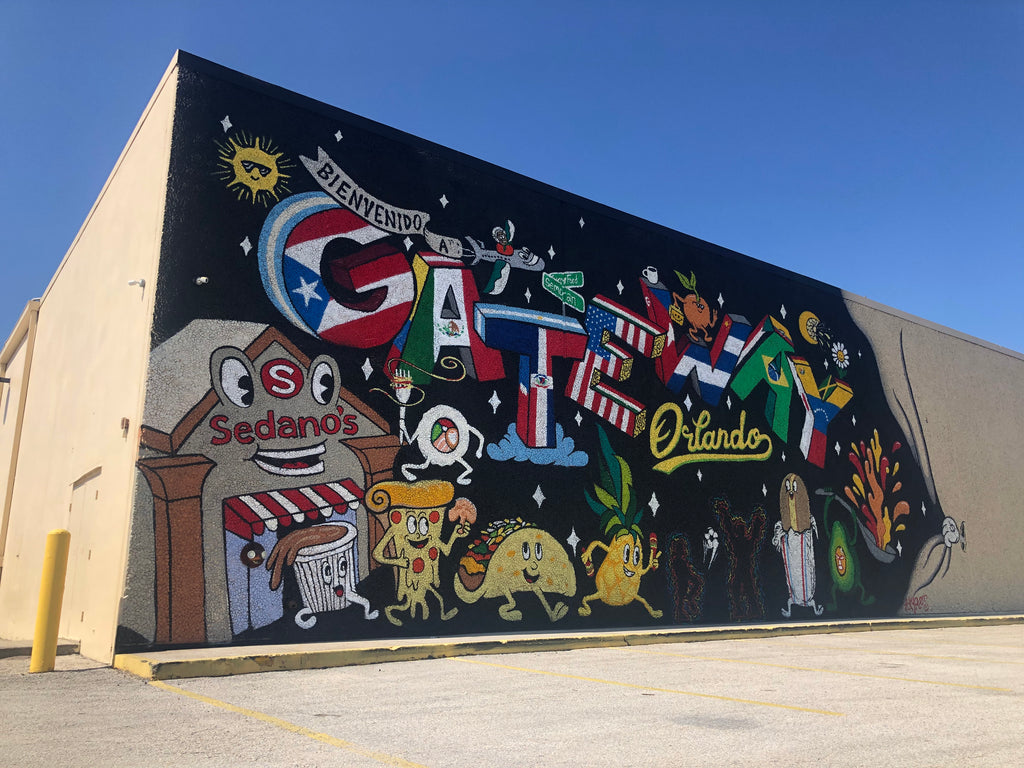The image depicts a vibrant mural on the side of a tan-colored building, captured in broad daylight with a bright cornflower blue sky in the background. The mural, located in a city alleyway near a parking lot, prominently features the word "Gateway" painted in large, fun capital block letters. Each letter is designed with different flags from around the world, including those of Mexico, the United States, Brazil, Puerto Rico, and Colombia. Above the word "Gateway," a banner reading "Bienvenido a" is being towed by a plane, accompanied by a smiling sun. Below the colorful lettering, the word "Orlando" is written in flowing yellow cursive. The bottom section of the mural showcases an array of cartoon-like anthropomorphized foods and objects, such as a taco, pizza, pineapple, avocado, and trash can, all with friendly faces. A building labeled "Sedano's," which appears to be a local store, is also depicted with eyes and a smiling mouth. The mural's bright, playful design is enhanced by the appearance of the tan coloring being ripped away, revealing the vivid artwork beneath.